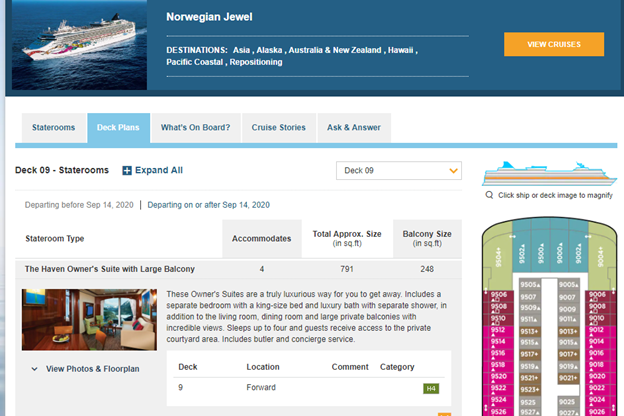The screenshot depicts a detailed view of a cruise webpage, specifically highlighting the Norwegian Jewel. In the top-left corner, there is a small square featuring an image of a cruise ship, alongside a blue rectangle labeled "Norwegian Jewel Destinations," listing various countries. An orange label to the side reads "View Cruises," albeit somewhat faintly. Below this section are five navigational tabs: Staterooms, Deck Plans, What's On Board, Cruise Stories, and Ask & Answer.

The majority-left side of the screen is dedicated to informative content, while the right side displays a side view image of the ship, each level represented in distinct colors. Below this image is a detailed map indicating cabin locations, color-coded with various hues such as bright magenta, pink, gray, brown in the center, turquoise at the top, and olive green on each side. To the left of the map, there is a descriptive paragraph offering more insights.